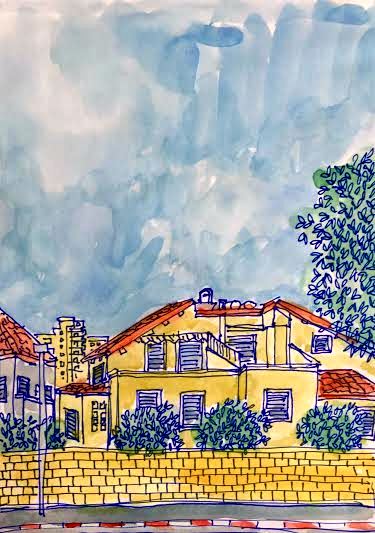In this detailed vertical watercolor painting, a vibrant, blue sky with subtle white clouds dominates the upper half of the image. Below the sky, a charming scene unfolds: a prominent yellow house with a distinctive Spanish-style orange clay tile roof catches the eye. The house features violet-colored shutters and is fronted by a yellow brick wall. 

To the right of the main house, a lush tree with green and violet foliage stands tall, rendered meticulously using pen and a green watercolor wash. In front of the house, four neatly aligned bushes share the same green and violet hues as the tree.

Adjacent and behind the central house, additional buildings in yellowish-orange tones with red-orange roofs suggest a bustling neighborhood or apartment complex. The scene includes a road marked with distinctive white and red stripes, enhancing the town-like feel. Gray window frames and a mix of gray and yellowish-orange pathways add to the structure and depth of the scene, evoking a picturesque morning in what appears to be a lively urban or suburban setting.